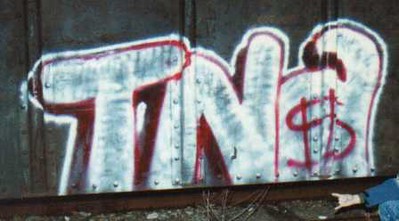The photograph captures a graffiti-covered metal wall, possibly an old railway car, characterized by visible steel bolts and a rusted red or brown surface. The focal point is the prominently spray-painted letters "T.N.A.," rendered in large white bubble letters with gray shading and a vivid red outline. Notably, the letter "A" features a red dollar sign at its center. In the lower right-hand corner of the image, a white cartoon hand, emerging from a blue sleeve, extends its index and pinky fingers in a devil horns or gang symbol gesture. Nearby, rusted rails and scattered rocks and sticks contribute to the gritty, industrial setting.